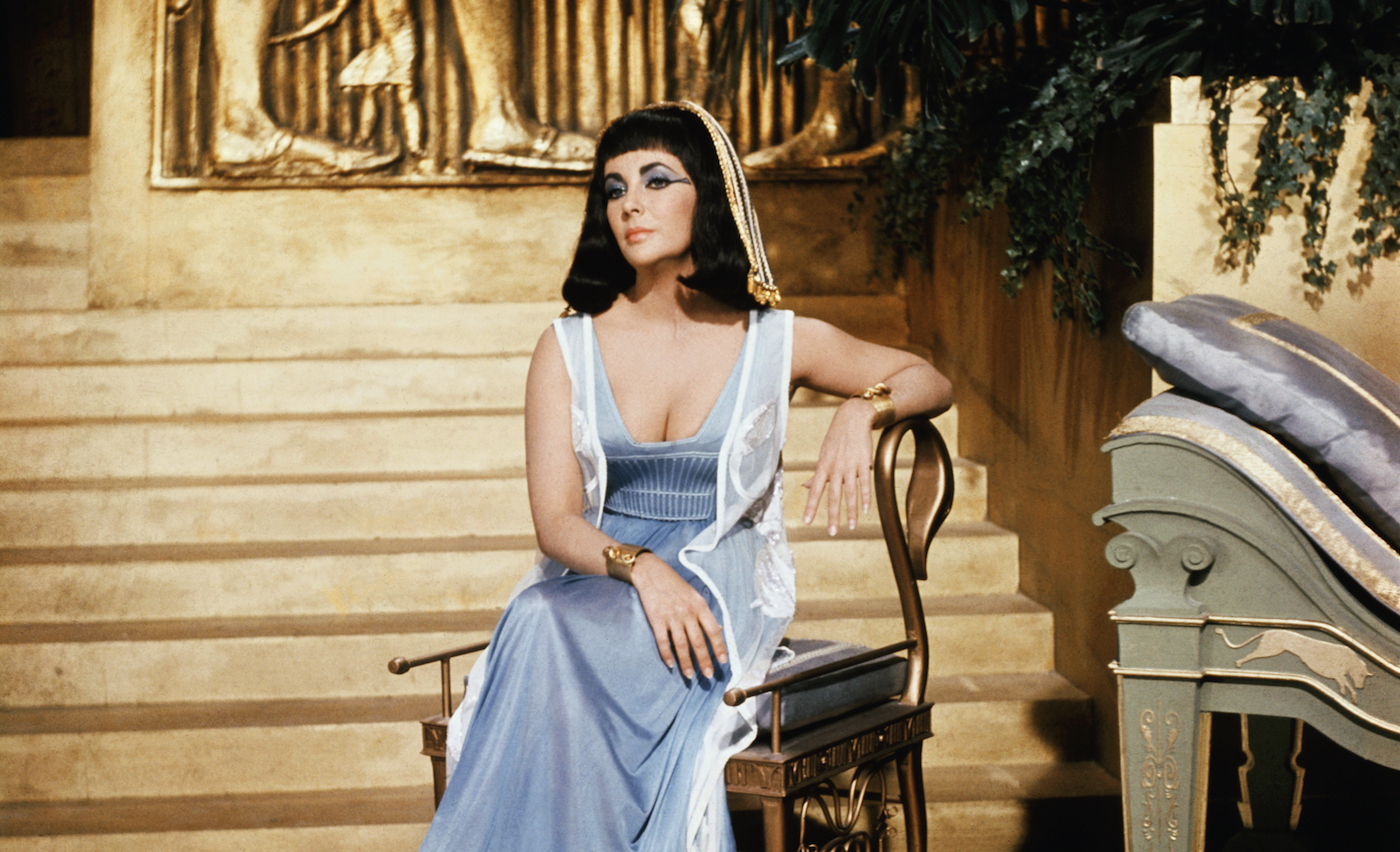In this evocative image, Elizabeth Taylor, portraying Cleopatra, captivates with her detailed attire and regal poise. Likely taken during her 30s or 40s, Taylor is adorned in a stunning blue dress with a low-cut neckline, complemented by a white vest overlay. Her wrists sparkle with thick gold bracelets, and her striking Cleopatra look is completed with a black shoulder-length wig with bangs, adorned by a white and gold beaded headdress. Her dramatic blue eyeshadow and prominent Egyptian-inspired eye makeup accentuate her legendary features.

Taylor is seated elegantly on a richly decorated, gold Egyptian-style chair, her arm resting casually on the armrest to the right of the image. The background is rich with historical ambiance, showing a series of steps leading up to a wall adorned with ancient relief sculptures, though only the feet and lower legs of these carvings are visible. To the right of the composition, an upholstered sofa or lounge chair is partially visible, distinguished by a blue pillow and flanked by lush plants. This scene beautifully combines elements of ancient Egyptian luxury with a portrait of a Hollywood icon in one of her most memorable roles.